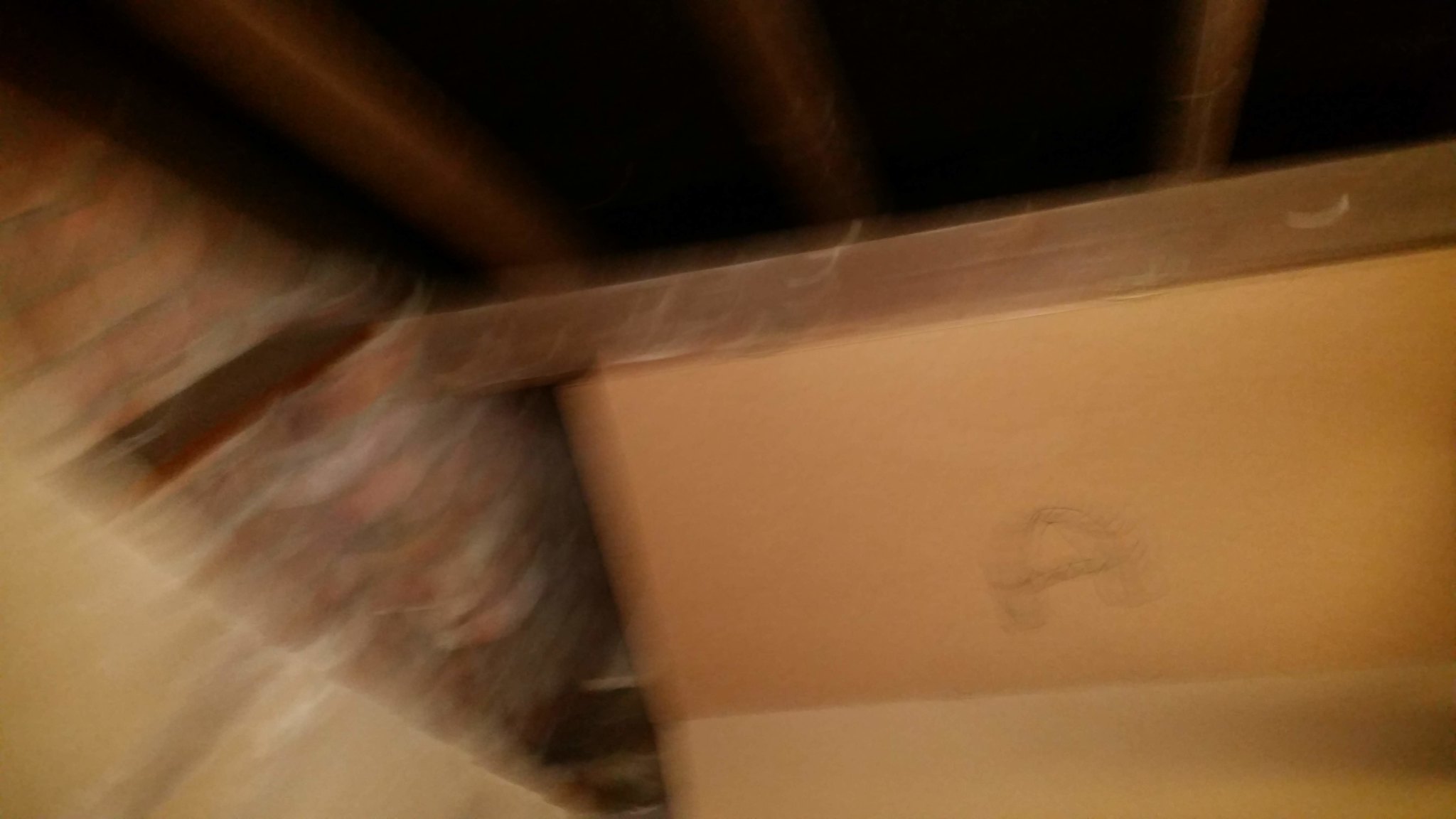This is a very blurry close-up photograph of a cluttered attic. To the left, a section of red, tan, and dark brown brick appears knocked out, partially covered by blurred tan-colored cardboard. The right side features more cardboard, with the top piece exhibiting a faded black drawing. The lower part of this cardboard is a light brown or tan color without any scribbles. Beside the cardboard, a dark gray board with light gray fading and scratches, along with a noticeable white gouge, is visible. Further to the right, a set of brown beams shows white scratches and gouges, characteristic of attic joists supporting a pointed roof. The movement implied by the blurriness suggests the photograph may have been taken inadvertently. There also seems to be an open cardboard box visible in the attic's dim lighting.